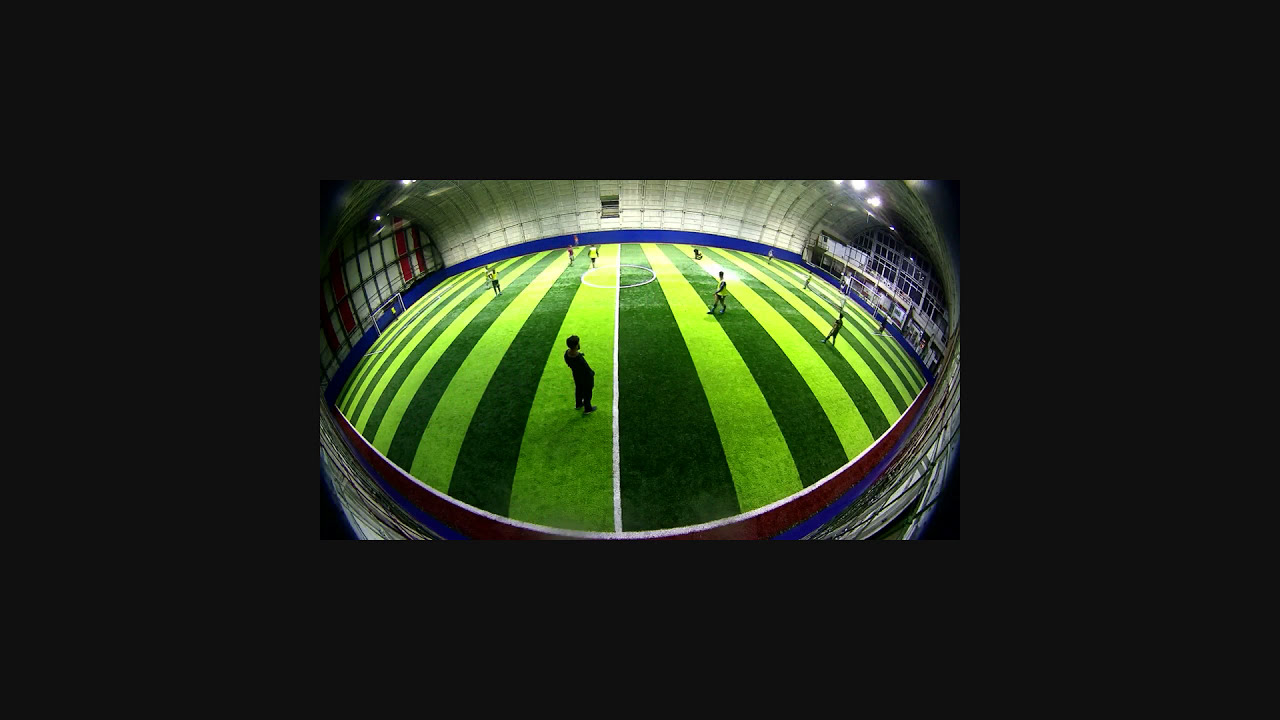The image captures a distorted, panoramic view of an indoor soccer field. The field, centered in the image, features alternating dark green and light green stripes, resembling a soccer field but with a bulging, rounded appearance as if viewed through a backward magnifying glass. The periphery of the field is enclosed by blue barriers that transition to red on the outside, with white walls curving inward to form a partial roof. Along the sides, scattered players in bright yellow jerseys are visible, standing sporadically around the field. White soccer goals are positioned on both the left and right sides, each situated below windows or smaller wall sections. The entire scene suggests a recreational indoor soccer game, emphasized by the absence of bleachers and the intimate, enclosed space.